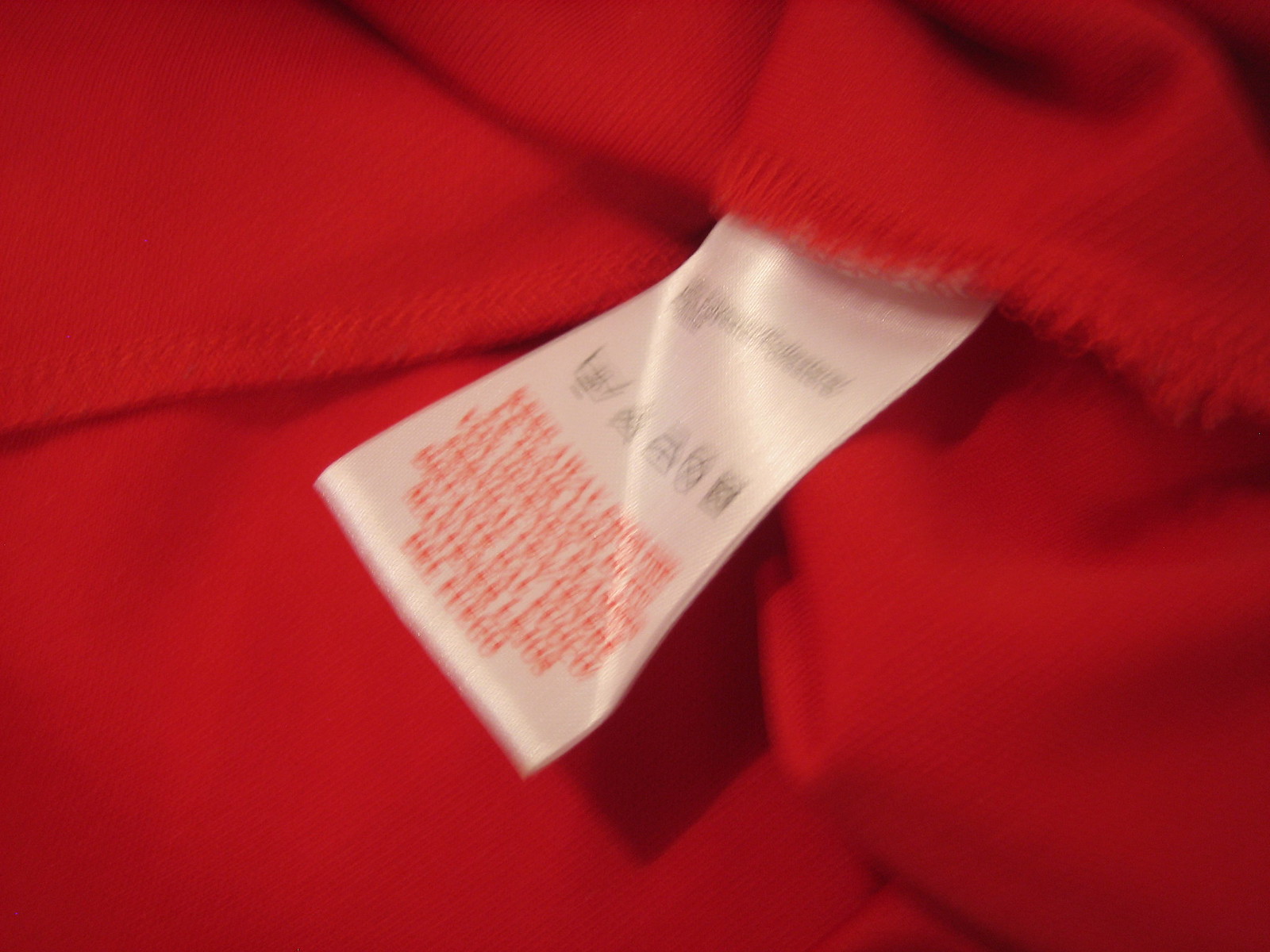The photograph depicts a red piece of fabric, potentially a clothing item, with the top edge folded over. Detailed red stitching runs horizontally across the top, with a visible frayed and slightly unraveled section on the upper right. Extending from the upper right corner is a white rectangular tag. Although the tag is too fuzzy to decipher completely, it contains black text at the top that is unreadable, followed by a series of images likely indicating care instructions for the item. Below these images, a cluster of red text presumably provides further washing instructions and material composition details. The overall image is blurred, making it challenging to read the finer details on the tag.